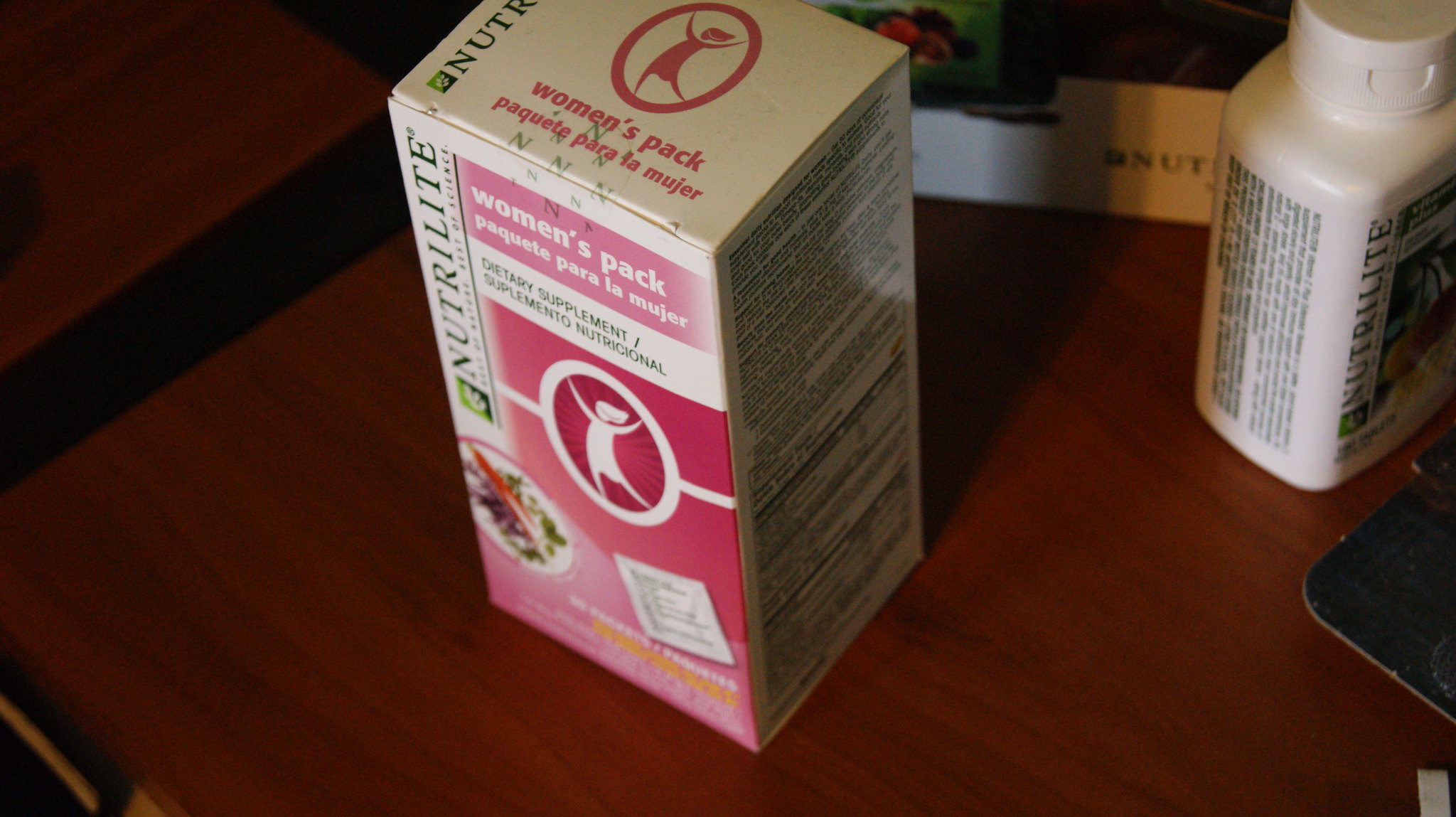The photograph captures a tabletop scene within a home, featuring several Nutrilite products prominently. The main item, positioned slightly to the left of center, is a white package with a pink front design. This package showcases a joyful female character with arms raised and one leg kicked back. The brand name "Nutrilite" is displayed in black lettering on a white background above the words "Women's Pack" written in white on the pink section, and "Dietary Supplement" printed in black. Additionally, the package includes multilingual labels, with "Paquete Para La Mujer" and "Suplemento Nutricial" also noted. On the bottom left corner of the package, there appears to be an image of possibly a salad with chopsticks, although it's somewhat ambiguous. The seal on this package, bearing a logo with an ‘N’, is still unbroken, indicating it hasn't been opened.

Adjacent to this, on the right side of the image, there is a noticeable white bottle, also by Nutrilite. The bottle is partially cast in shadow, making it difficult to discern specific details about its label. The tabletop itself is made of medium red-brown wood, adding a warm tone to the setting. Behind the main package, there’s another Nutrilite box, also white, visible in the background. In the lower right-hand corner, the edge of a black cell phone can be seen, resting on the table. This detailed composition clearly highlights the Nutrilite Women's Pack and related products within a homey environment.